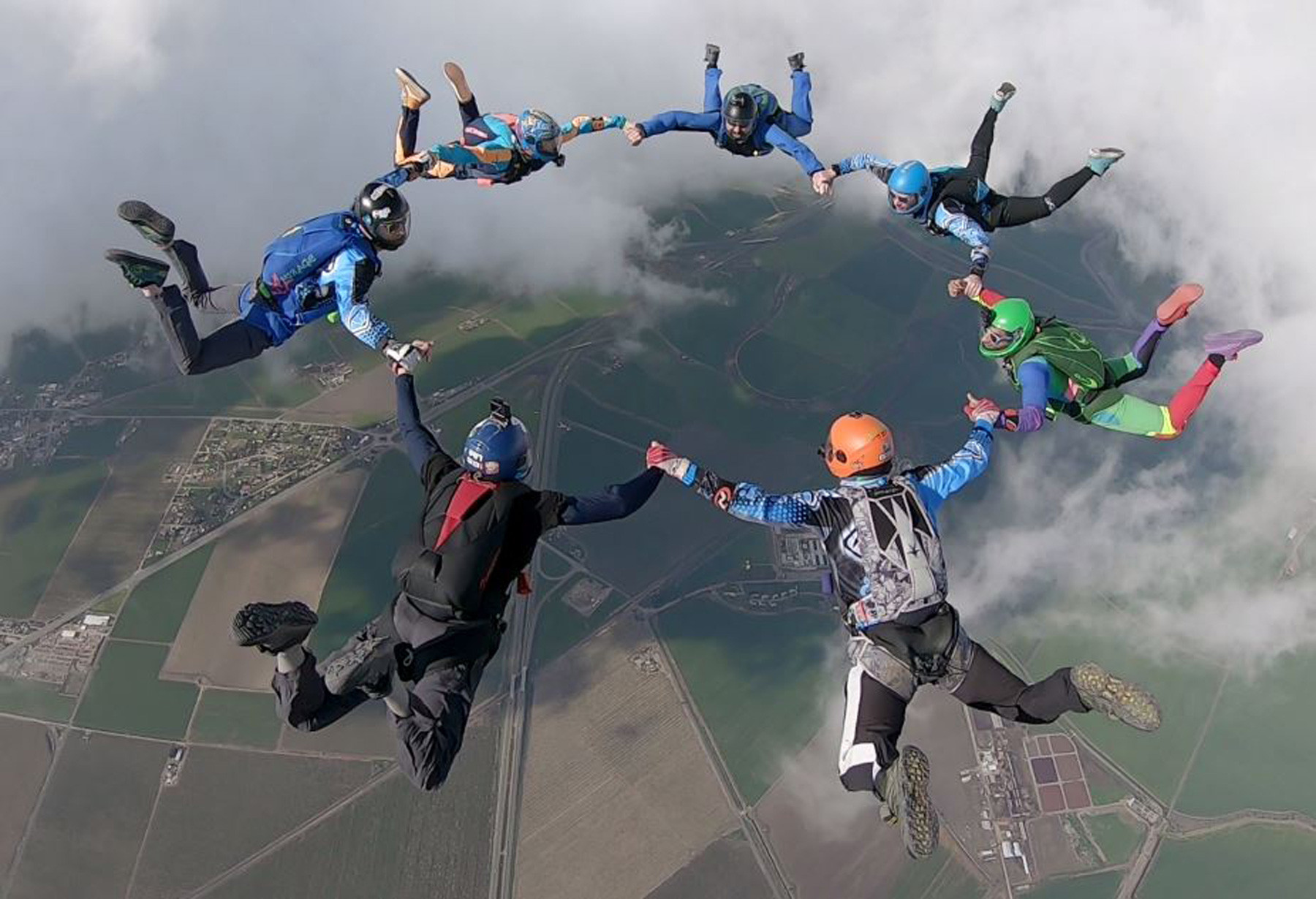A breathtaking aerial shot captures seven skydivers, all wearing parachute backpacks and helmets, forming a circle mid-air while holding hands. Each skydiver sports different colored gear, including helmets in shades of blue, black, green, and orange; some even have GoPro cameras attached. The group appears to be roughly five to six thousand feet above the ground. The landscape below reveals a patchwork of green fields, some buildings, houses, and distant roads, while fluffy clouds still surround them, especially at the top of the image. The scene is exhilarating and slightly intimidating, as the group, likely photographed by another skydiver from above, prepares to deploy their parachutes soon.